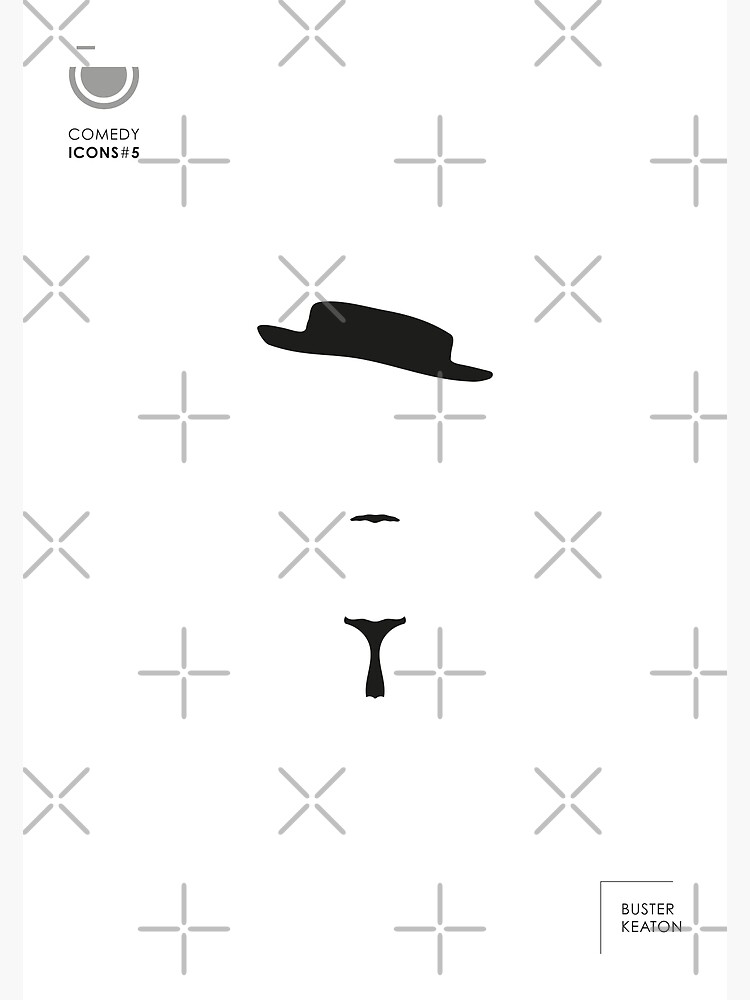The image features a white background adorned with an evenly distributed pattern of gray X's and crosses. Starting at the top, three gray X's are aligned horizontally, with precise spacing of about two inches between each. This pattern continues vertically down the page, alternating with rows of plus signs (crosses) directly beneath the X's. In the top left corner, a gray circle encases the text "Comedy Icons #5." Dominating the center of the image is a stylized representation of Buster Keaton, comprising a slightly tilted black hat, a black mustache positioned below it, and a black tie, all rendered as solid shapes against the background. This iconic attire stands in stark contrast to the surrounding pattern. In the bottom right corner, a partially bordered rectangle frames the text "Buster Keaton," with only the top and left sides of the border visible, keeping the presentation minimalist and focused. This structured yet simple arrangement suggests a tribute to the silent film legend through a blend of graphic design and thematic elements.